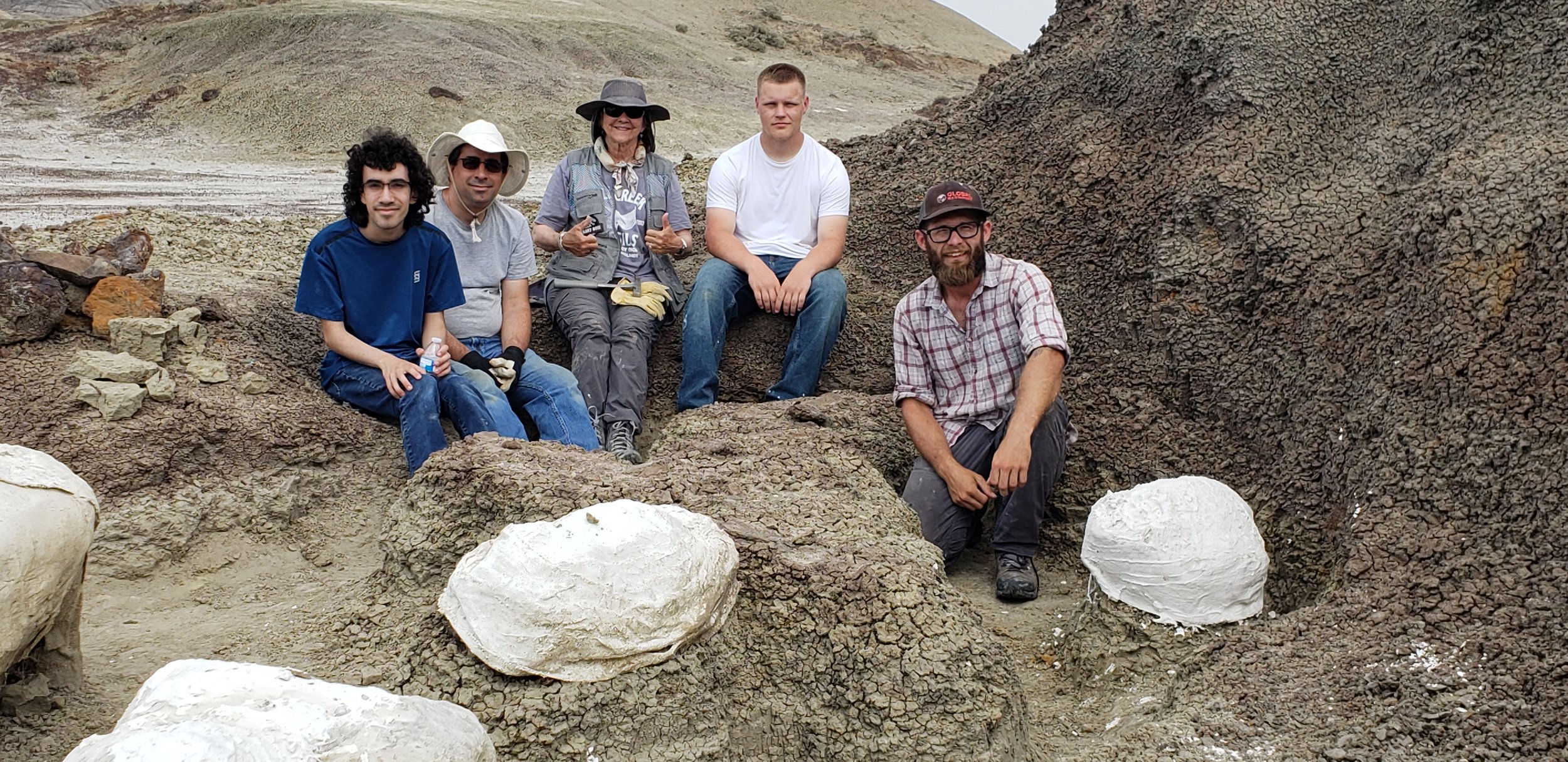The image is a detailed color photograph of an archaeological dig site. The surface is a dried, cracked mud or dirt, typical of a desert environment. In the scene, five scientists—four men and one woman—are gathered around a pit they have been excavating. The group appears cheerful, posing with several large white plaster-covered objects, possibly fossils or significant finds, arranged near them.

To the right of the image, one man is crouched with a brown baseball cap, black-rimmed glasses, a red and blue checkered button-up shirt with rolled-up sleeves, gray pants, and tennis shoes. Nearby, another young man in a white sleeveless shirt and blue jeans is seated on a rock. The woman in the group, positioned centrally, is wearing a gray vest, a bluish-gray shirt, jeans, a gray digging-style hat, and sunglasses while giving two thumbs up. Another man in a gray shirt, jeans, and a similar hat sits beside her. The fifth person, a younger teenager with curly black hair and glasses, is sporting a blue shirt and jeans.

Behind them, varying shades of tan and brown hills and a steeper dirt hill featuring scrubby brush reveal the rugged terrain. A semi-visible road in the background indicates the site’s accessibility. Strewn around the pit are rocks and gravel, with some stacked atop each other, and the overall atmosphere suggests these scientists have been diligently working on their excavation.